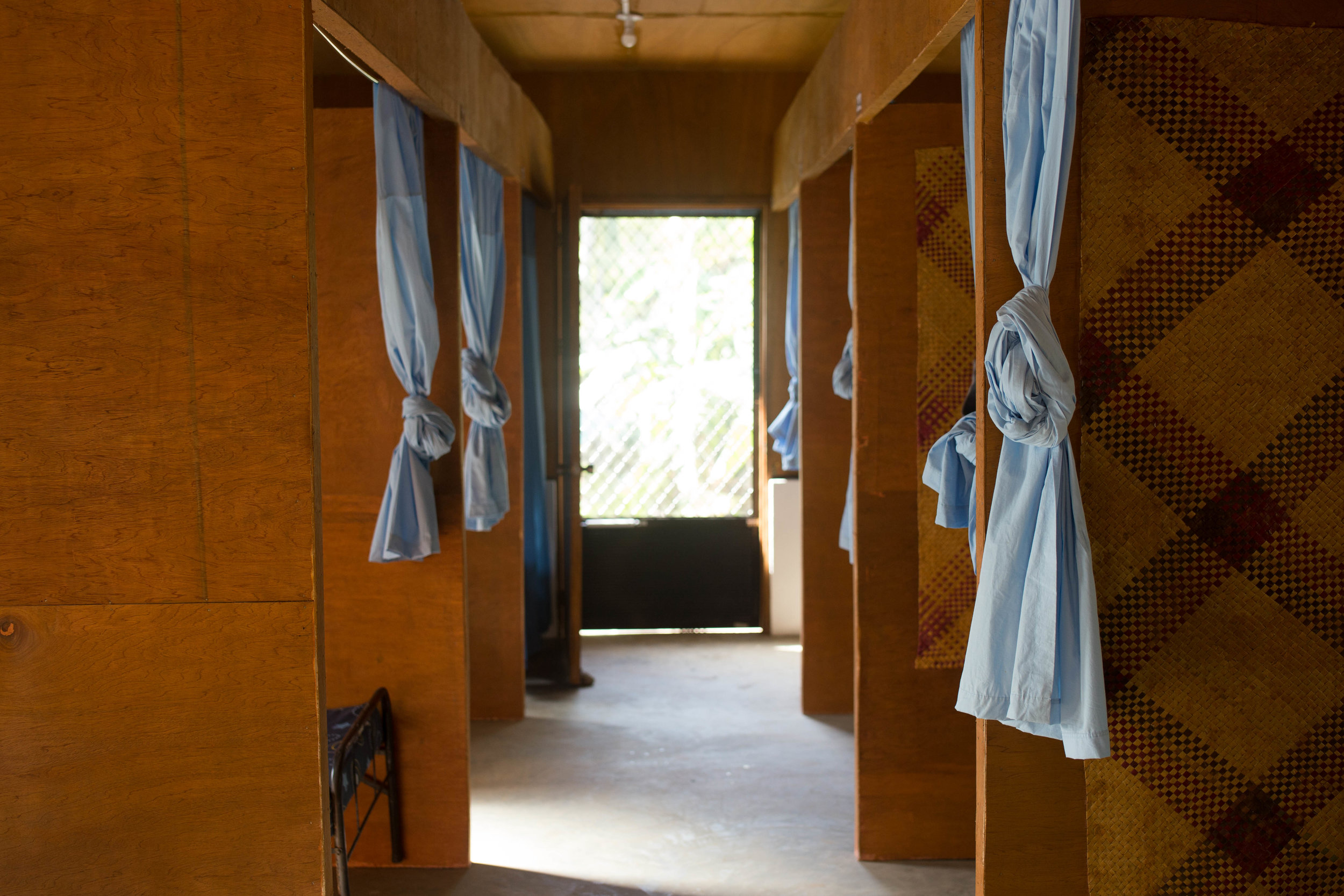The image depicts a long, narrow hallway within a rustic wooden structure, possibly located in a third world country. The hallway extends towards an open doorway at the center of the image, beyond which a window is faintly visible. The building appears to be constructed from light brown wood, accentuated by several private compartments on either side of the hallway. There are seven compartments in total—three on the left and four on the right—all separated by curtains that are tied in knots, hanging halfway down. The curtains are light blue in color, adding a modest touch of vibrancy to the otherwise earthy palette that includes shades of brown, gray, blue, black, green, and white.

Inside the first compartment on the left, a black metal bed frame is visible, while a chair protrudes into the hallway, hinting at limited space. The compartments on the right feature a distinctive crosshatched diamond pattern in dark brown. This setup provides minimal privacy, hinting at the possibility of the space being used for dressing rooms or simple bedrooms. The floor is a flat, light gray surface, the material of which is indeterminate. Above, a basic LED or incandescent light fixture casts a modest glow over the scene, contributing to the simplistic and austere ambiance of the setting.